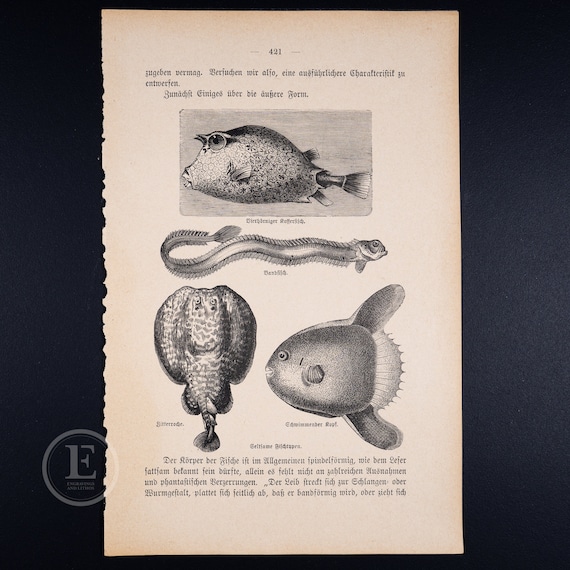This image captures an old, yellowish-brown page numbered 421 from a book of sea creatures, lying on a plain black surface. The page features detailed black-and-white illustrations of four different marine animals. At the top is a prehistoric-looking puffer fish with big eyes, speckled patterns, and small fins, facing left. Below it, centered on the page, is a long, slender eel-like creature, facing right and appearing about 25% longer than the puffer fish. At the bottom are two more illustrations: on the left, a creature resembling a stingray, and on the right, an undistinguishable fish with fins on its top and bottom, facing left. The text on the page is too small to read and appears to be in a different language, possibly providing information about each creature. The edges of the page are slightly serrated, as if torn from the book, and there is an "E" stamp in a circle partially overlaying the background image. The entire scene rests against the stark contrast of the black surface, enhancing the vintage feel of the yellowed page and its intricate illustrations.